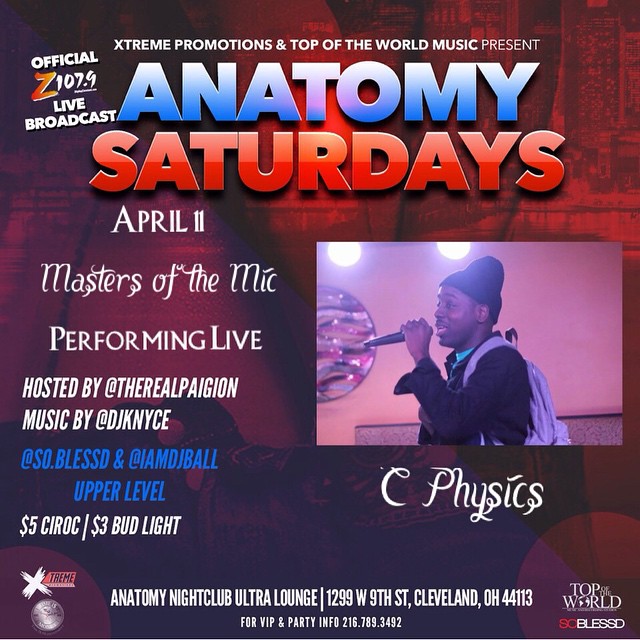This is a flyer for an upcoming event at Anatomy Nightclub Ultra Lounge. The background features a dark red and purple gradient design, possibly inside a building. Dominating the top center in large block letters, it reads "Anatomy Saturdays." "Anatomy" is in blue with white tips, and "Saturdays" is in red with a lighter shade on the upper part. Beneath this, the flyer announces "April 11th" and "Masters of the Mic performing live," followed by host details: "Hosted by The Real Pagan" and "Music by DJK Nice NYCE" in white text.

On the left, more details continue in blue text: "@SoBlessed and @IMDJBall upper level." Further down in white text, it mentions "$5 Ciroc, $3 Bud Light." Centered at the bottom, it reads "Anatomy Nightclub Ultra Lounge, 1299 West 9th Street, Cleveland, Ohio, 44113," with small text below it for VIP and party info: "216.789.3492."

In the middle right section, there is a square image of a man, labeled as "C. Physix." He is viewed from his left side, holding a microphone to his mouth, and appears to be singing. He wears a black beanie, a black long sleeve top, and a backpack. The flyer also states "Extreme Promotions and Top of the World Music Present," with a mention of it being an official "Z107.9 live broadcast" and "Top of the World" in the bottom right corner.